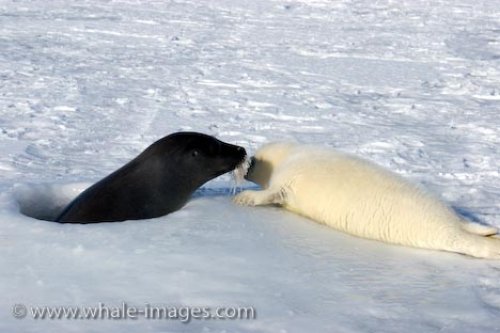This captivating photo from www.whale-images.com, prominently watermarked in white in the bottom left corner, captures a serene yet striking moment in a frozen, tundra-like landscape. At the center of the scene, a pristine, perfectly round hole in the ice commands attention. Emerging from this hole is a black seal, its head and whiskers visible as it appears to engage with a nearby white baby seal. The black seal faces the right, its gaze fixed on the young seal, whose fluffy fur indicates its very recent birth. The white seal lies flat on its belly on the ice, facing away from the camera, adding a tender contrast against the wintry backdrop. The scene is bathed in the quiet stillness of the arctic environment, punctuated by these two creatures' intimate interaction.